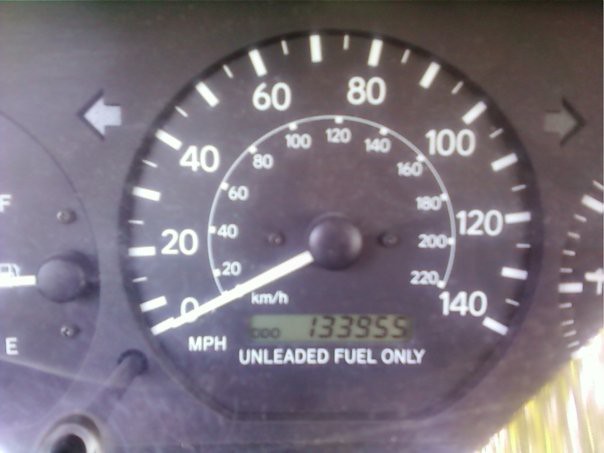A close-up view of a car's speedometer predominantly features a sleek black background with crisp white markings and numbers. The speedometer indicates a current speed of 0 mph, signifying that the vehicle is stationary. Below the speedometer, a digital odometer displays an impressive reading of 133,955 miles. Directly beneath this, the phrase "UNLEADED FUEL ONLY" is clearly visible in white lettering. To the left, a partially visible fuel gauge shows that the fuel level is at approximately half a tank. An intriguing visual effect is present in the lower right corner, where a glare or reflection, resembling the view of sunlight filtering through blades of grass, forms a triangle, adding an interesting dynamic to the image.